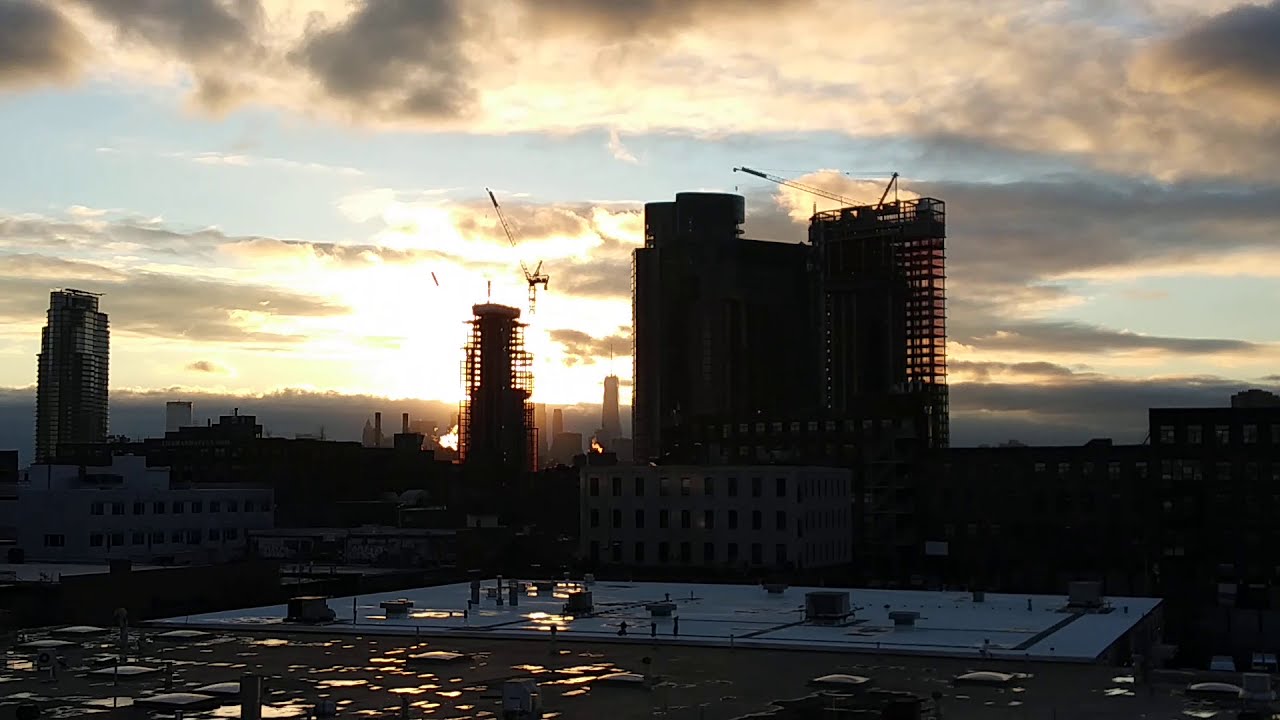This photograph captures a cityscape at either sunset or sunrise from a rooftop perspective. The scene is bathed in the soft, diffused light of the sun poking through gray and white clouds, casting the skyline into shadowy relief. Among the buildings, you can see a few under construction, identifiable by the large cranes perched on or beside them. The horizon is dotted with both completed and half-built structures, creating an industrial yet picturesque panorama against a backdrop of blue skies with scattered clouds. In the foreground, a darkened, flat rooftop anchors the image, with the buildings and their countless windows stretching out towards the horizon. The overall palette combines muted tones of black, light blue, gray, white, and hints of yellow, emphasizing the twilight atmosphere.